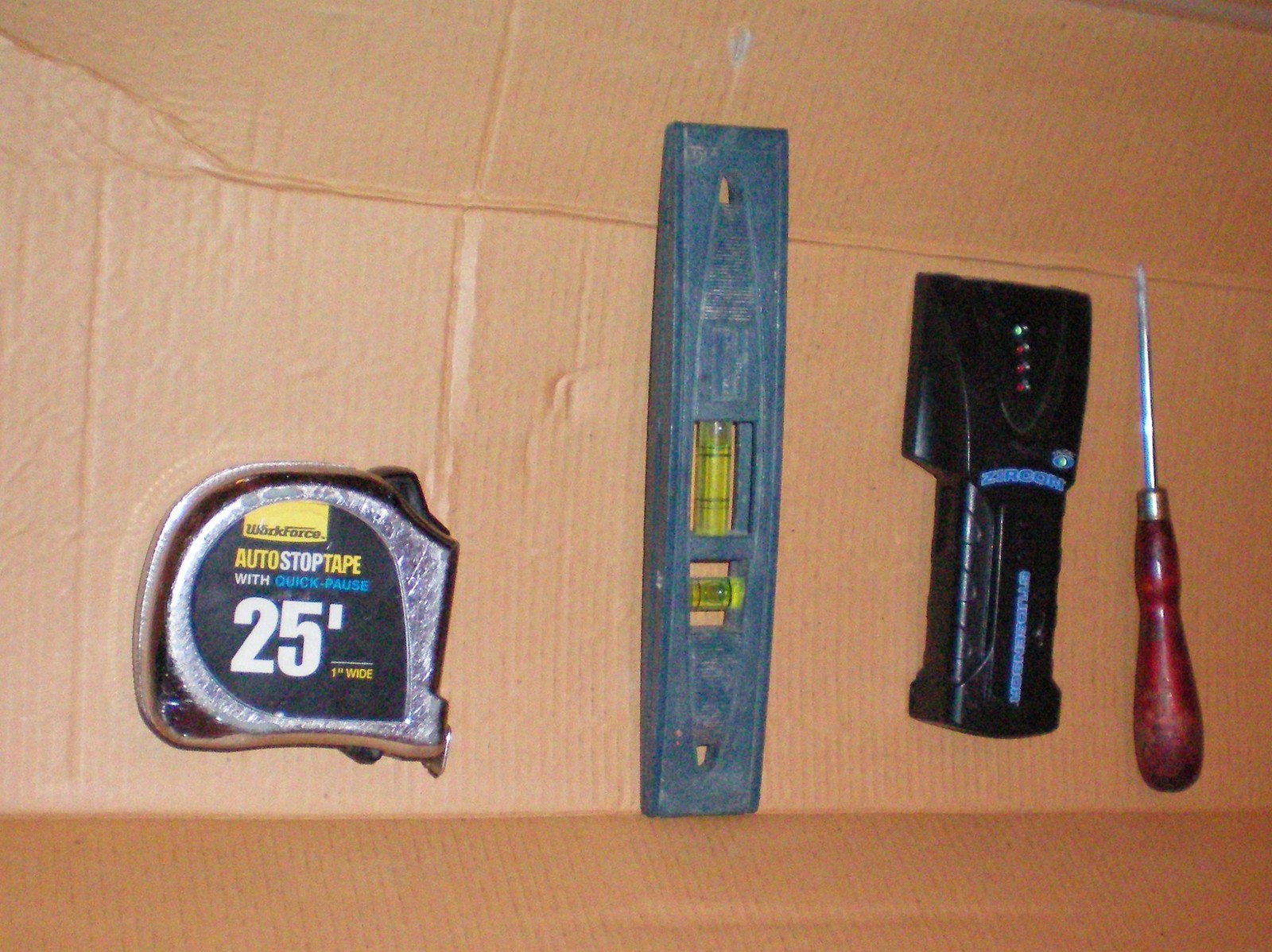The image displays four commonly used household tools meticulously aligned in a horizontal row on a deconstructed piece of cardboard. From left to right, the first tool is a 25-foot-long tape measure housed in a silver metallic casing, adorned with a label that reads "Workforce Auto-Stop Tape," featuring a 1-inch-wide measurement. Next in line is a blue spirit level with a vibrant neon yellow-green liquid-filled tube, used for determining the level accuracy of surfaces. The third tool is a black stud finder, featuring blue branding and four indicator lights—three red and one green, designed for locating studs in walls. Lastly, there is a red-handled screwdriver with a metal tip, its handle exhibiting a wooden appearance with darker accents and a gold-colored band at the base. All four tools rest on the cardboard surface, providing a comprehensive display of essential home improvement instruments.